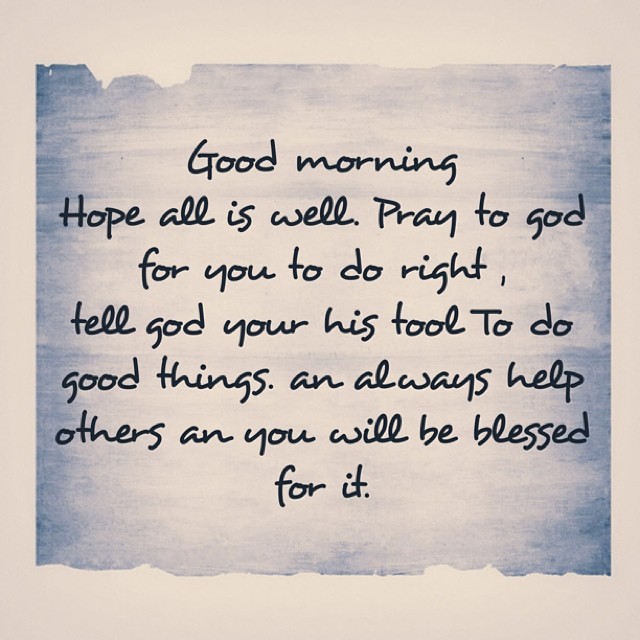This square-shaped image features an inspirational quote crafted to resemble a handwritten note, making it ideal for framing or display on a webpage. The note, seemingly worn and slightly torn along the edges, is set against a softly washed blue and white watercolor-like background. Its black, handwriting-style font delivers a heartfelt message: "Good morning. Hope all is well. Pray to God for you to do right. Tell God you're His tool to do good things and always help others and you will be blessed for it." The note appears to be laid on a white surface, creating a natural border around the blue-tinged paper, giving it a warm, personal touch.